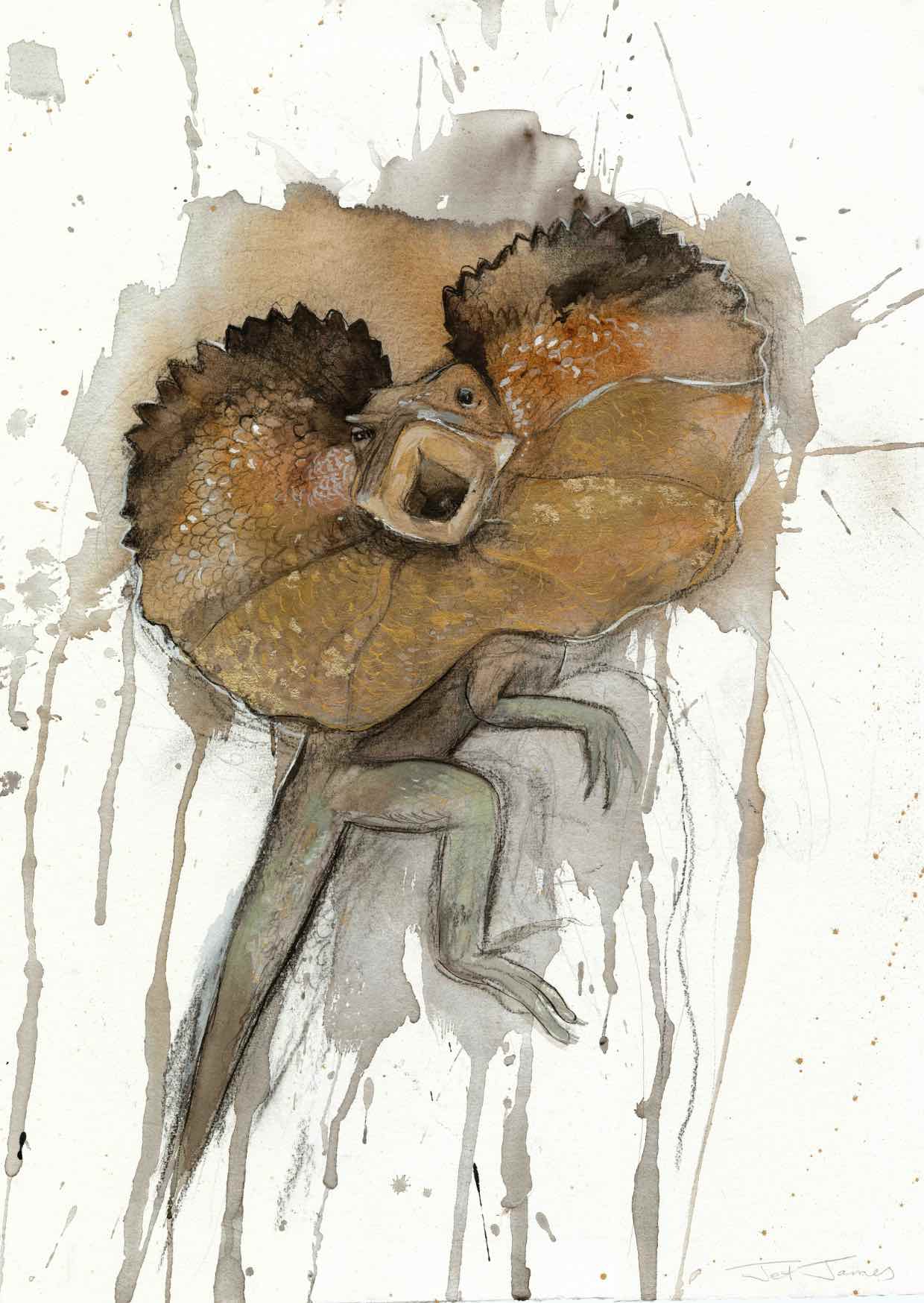The artwork is a rectangular, vertical watercolor painting featuring an abstract representation of a frilled lizard. Set against a predominantly white background, the painting depicts the lizard in a horizontal-oval shape, subtly tipped diagonally. The lizard's head, adorned with a detailed, frilled neck resembling inflated skin, dominates the composition. The head and frill showcase intricate lines depicting veins, fringed edges, and small white circular accents, with the eyes and open mouth clearly visible. The head is primarily brown, green, and gray, and contrasts against the less detailed, grayish-white body, which appears to be lying down or clinging to a surface. Dripping paint lines cascade from the body, as though connecting the lizard to the background, enhancing the abstract nature of the piece.